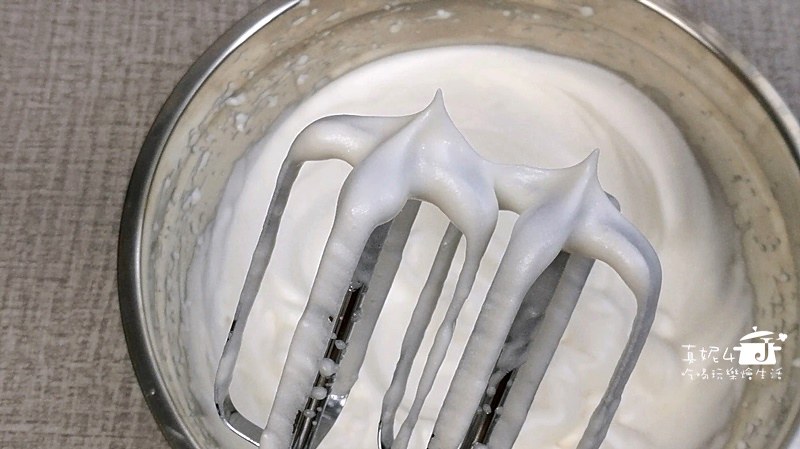A detailed photograph showcases a glass bowl brimming with thick, white whipped cream or meringue, poised on a tablecloth adorned with a varied design and a dark crisscross pattern. Above the bowl are two four-bladed interlocking beaters, likely from a hand mixer, made of silver metal with their central shafts coated in the same creamy substance. The beaters, one still attached to the mixer, exhibit perfect peaks formed from this whipped consistency, signaling that the mixture is thick yet smooth. The bowl's glass gleams, reflecting edges of stainless steel, adding depth to the scene. In the bottom right corner of the image, there is Asian writing alongside a stock pot with its lid slightly ajar, marked by a capital letter 'J'.